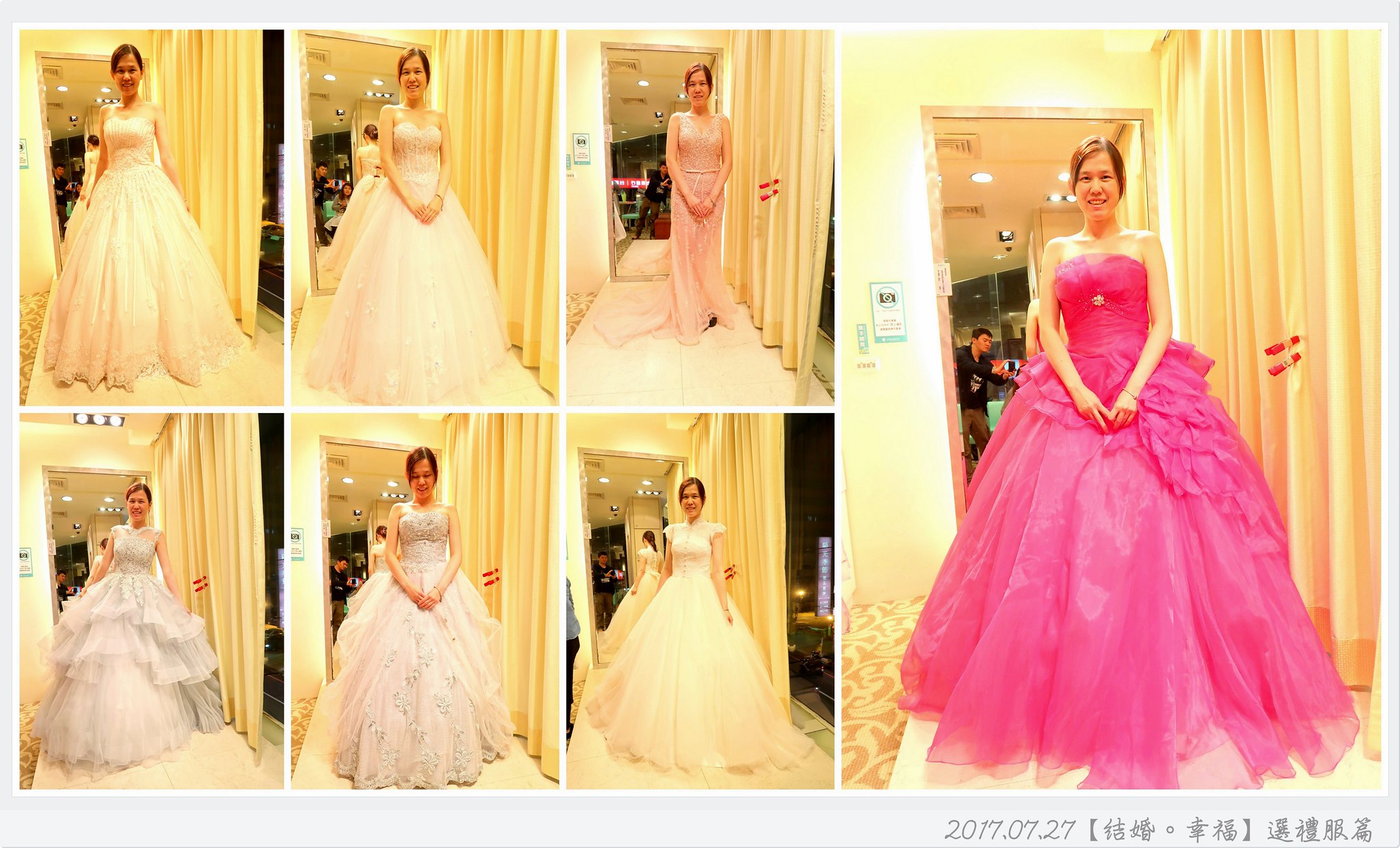The image features a series of seven photographs of an Asian woman with light brown hair pulled back, showcasing various outfits. There are six smaller photos arranged in a 2x3 grid on the left, and a larger photo to the right. The smaller photos all depict the woman modeling different wedding dresses, with three in bright white, two in different shades of white, and one in an off-white jumpsuit. The larger photo shows her in a vibrant fuchsia pink dress. In all the photos, she stands in front of shades and a window, with a mirror visible behind her. At the bottom of the image, the date "2017-07-27" is displayed, accompanied by some Asian characters. The arrangement suggests that the images were taken to help her choose a dress, likely for a wedding.